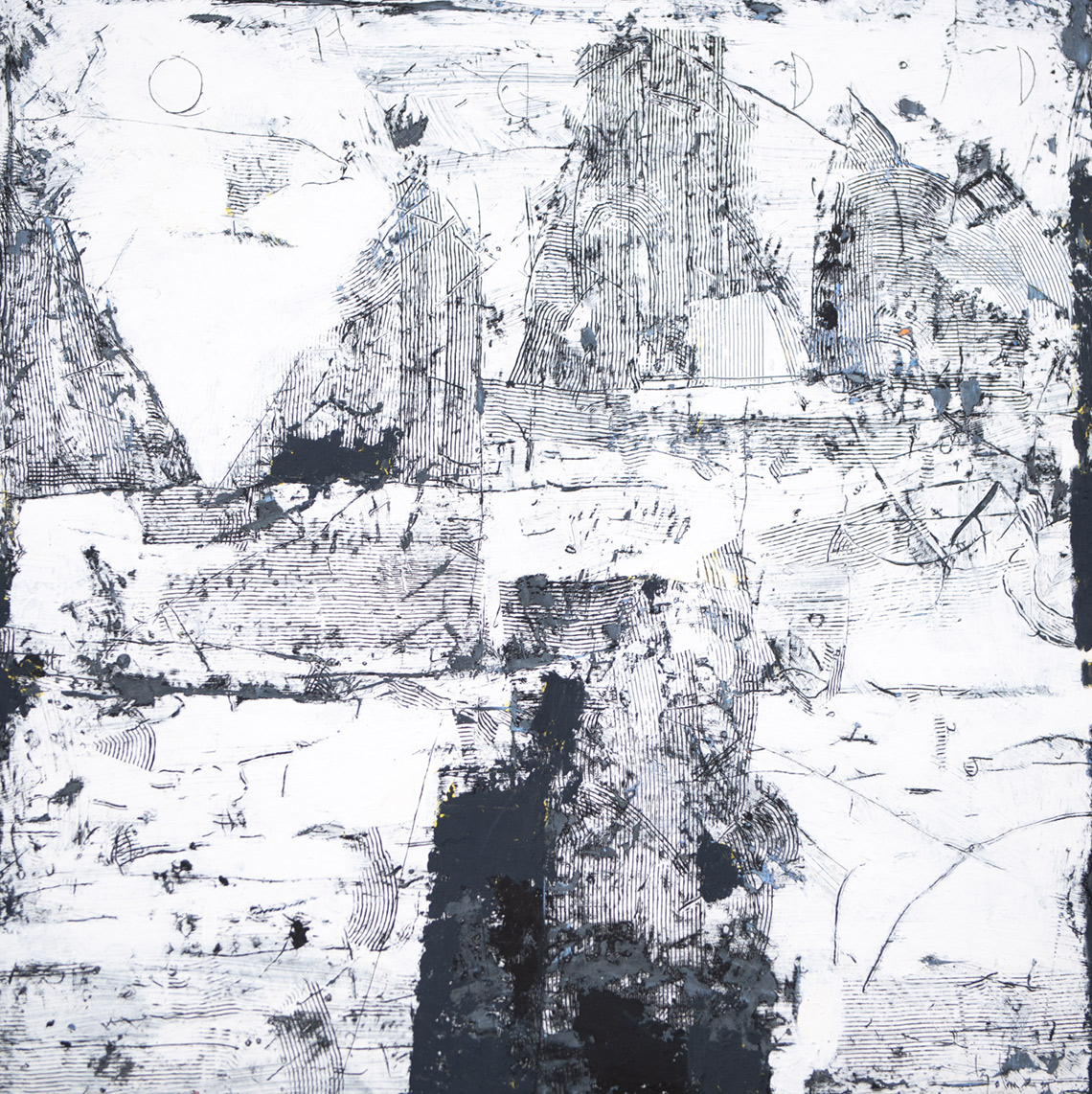The image is a black and white abstract artwork, seemingly created with black ink or paint. It features a chaotic array of lines—a mixture of horizontal, vertical, and curved strokes—and scattered splotches that vary in intensity. The most prominent dark area is located at the very center bottom, where the black appears densely applied and begins to lighten away from this point. Within the seemingly random composition, there are some discernible shapes: a couple of circles and half-circles, with a notable round outline in the top left corner. The artwork lacks a frame and gives an impression of visual disorder, somewhat resembling glue patterns under old floor tiles or an abstract rendering of sailboats. Despite its chaotic appearance, the piece is a study in contrast and form, composed entirely in black and white.